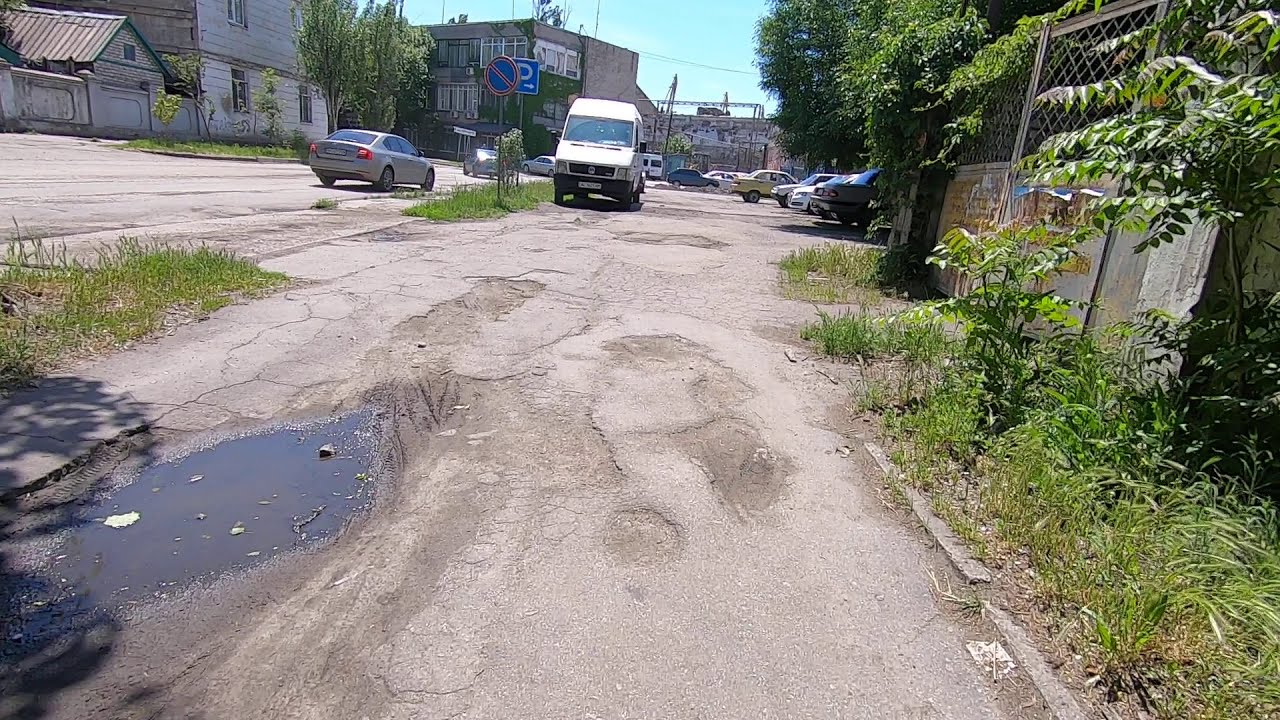The image depicts a somewhat weathered urban street scene with visible signs of wear and moisture. The asphalt is marred with water puddles and torn patches, suggesting recent rain or poor maintenance. On the left side of the street, a white van is parked, flanked by two blue signs—one indicating parking with an arrow to the right and another sign prohibiting parking, marked by a red circle with a dash through it against a blue background.

The street is divided into two lanes by a thin median of green grass and vegetation. Adjacent to the van and further left, a silver sedan is seen driving away from the viewer. In the immediate foreground on the bottom left corner, there’s a noticeable mud puddle, adding to the scene's gritty atmosphere.

To the right of the street, there's a half-brick, half-chain-link fence overgrown with green foliage and weeds. Beyond this, more cars are parked, suggesting proximity to a building or venue. The distant backdrop reveals a streetscape with multiple buildings: a weather-beaten brown building with an arched roof and peeling paint, an adjacent light-colored building that transitions from white at the bottom to gray at the top, and a further multi-story light brick structure filled with windows.

Farther in the distance, construction cranes jut into the light blue sky, hinting at ongoing development. The left side of the image is further characterized by a thick-leaved green tree and additional rundown structures, contributing to the overall ambiance of urban decay and renewal.